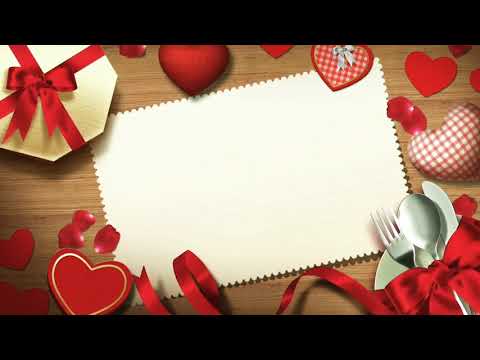The image depicts a cartoony, Valentine's Day-themed scene set on a wooden surface. At the center, there's a fancy white rectangle with scalloped edges, resembling a decorative piece of paper or stationery, serving as a blank space for writing. Surrounding the paper are numerous red hearts, some solid red and others with a red plaid pattern, as well as red rose petals and streamers.

In the top left corner, there's a heart-shaped box of chocolates, adorned with a red bow and suggesting a celebratory gift. The lower right corner features a place setting comprising a fork, knife, and spoon, tied together with a red ribbon. The entire composition, enclosed by two frames, exudes a festive Valentine’s Day atmosphere.